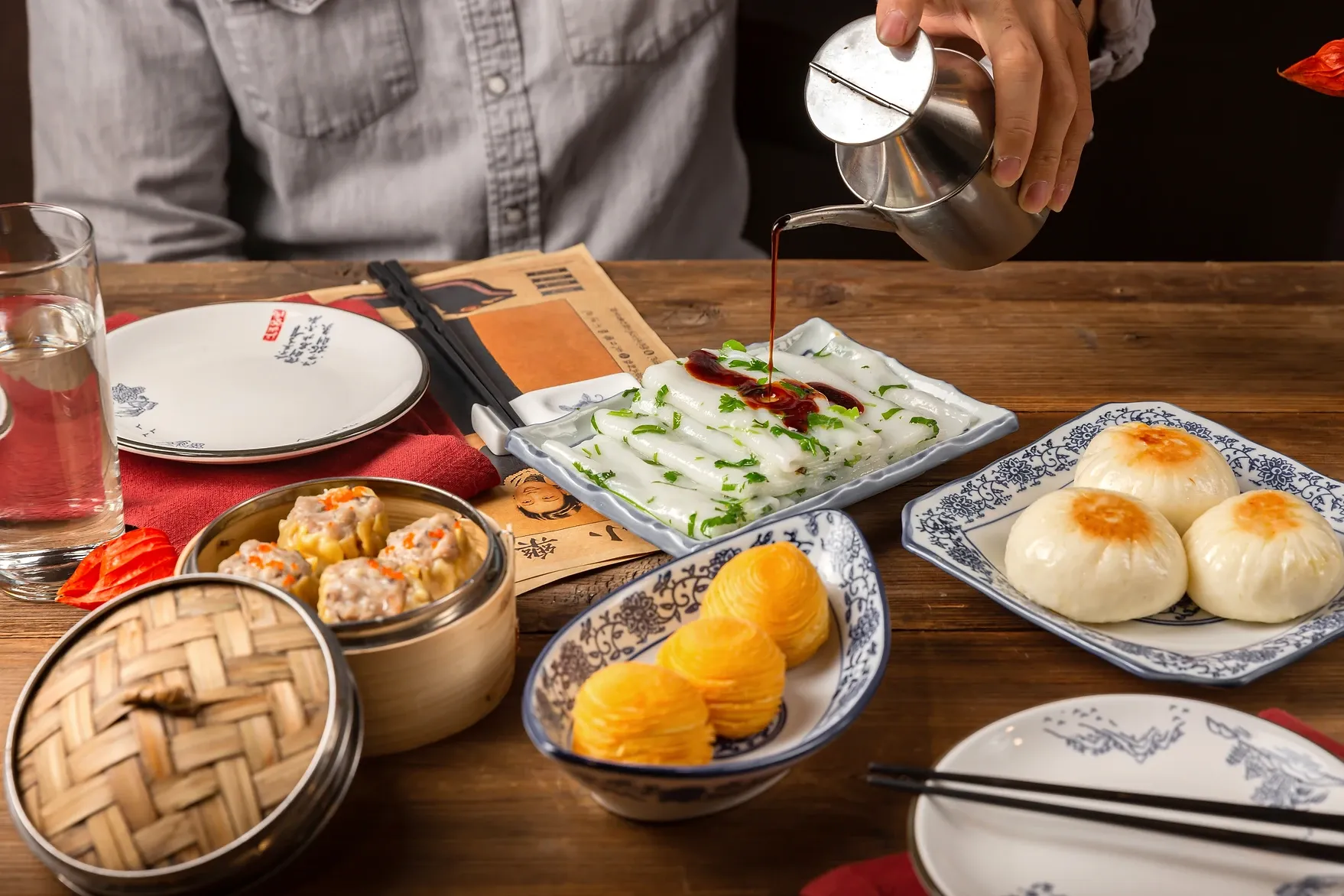This image features a wooden dining table set for a meal, prominently showcasing various Asian dishes, indicating a dim sum spread or Chinese breakfast. On the far right of the table, a glass of water, black chopsticks resting on a mat, and a neatly folded napkin accompany the place setting. To the left, a bamboo steamer contains four pork dumplings (shumai). Centrally placed is a blue and white bowl holding three orange items, likely dumplings or another small dish. Above that, a blue plate has white rice noodle rolls (chun fun) garnished with green chives, while a man wearing a grayish button-down chambray shirt is seen pouring soy sauce from a small teacup onto the rolls. A similarly patterned blue and white plate next to it holds three more dumplings—white with orange tops. There are also indications of other dishes, possibly steamed buns or pastries, completing the diverse array of dim sum offerings. The setup and the top-down angle of the photo give it an intimate, candid feel, capturing the essence of a casual dining moment.